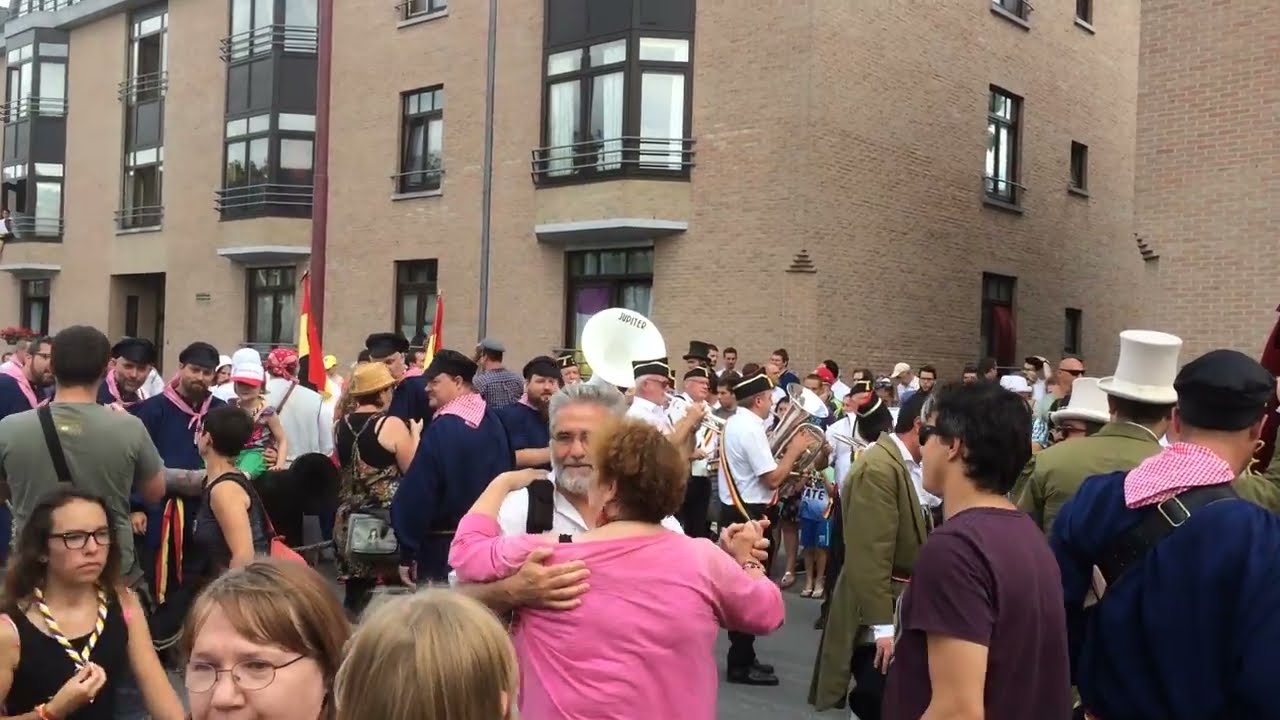In this vibrant outdoor city street scene, a lively festival is unfolding, complete with a bustling crowd and a marching band. The band members, dressed in coordinated outfits with white tops, black pants, and hats, parade through the street playing various musical instruments like tubas and trombones. Amidst the crowd, a man and a woman, the latter with red hair and a pink top, dance joyfully. There are other people with pink scarves tied around their necks and some wearing glasses. The background is dominated by imposing, tan-colored brick buildings with numerous windows and balconies, reaching up to the top of the image, contributing to the urban setting. A flag with red, yellow, and black stripes, possibly the German flag, is visible, hinting at a cultural or national celebration. People can be seen engaging in different activities—walking, talking, and laughing—adding to the festive atmosphere of this lively parade.